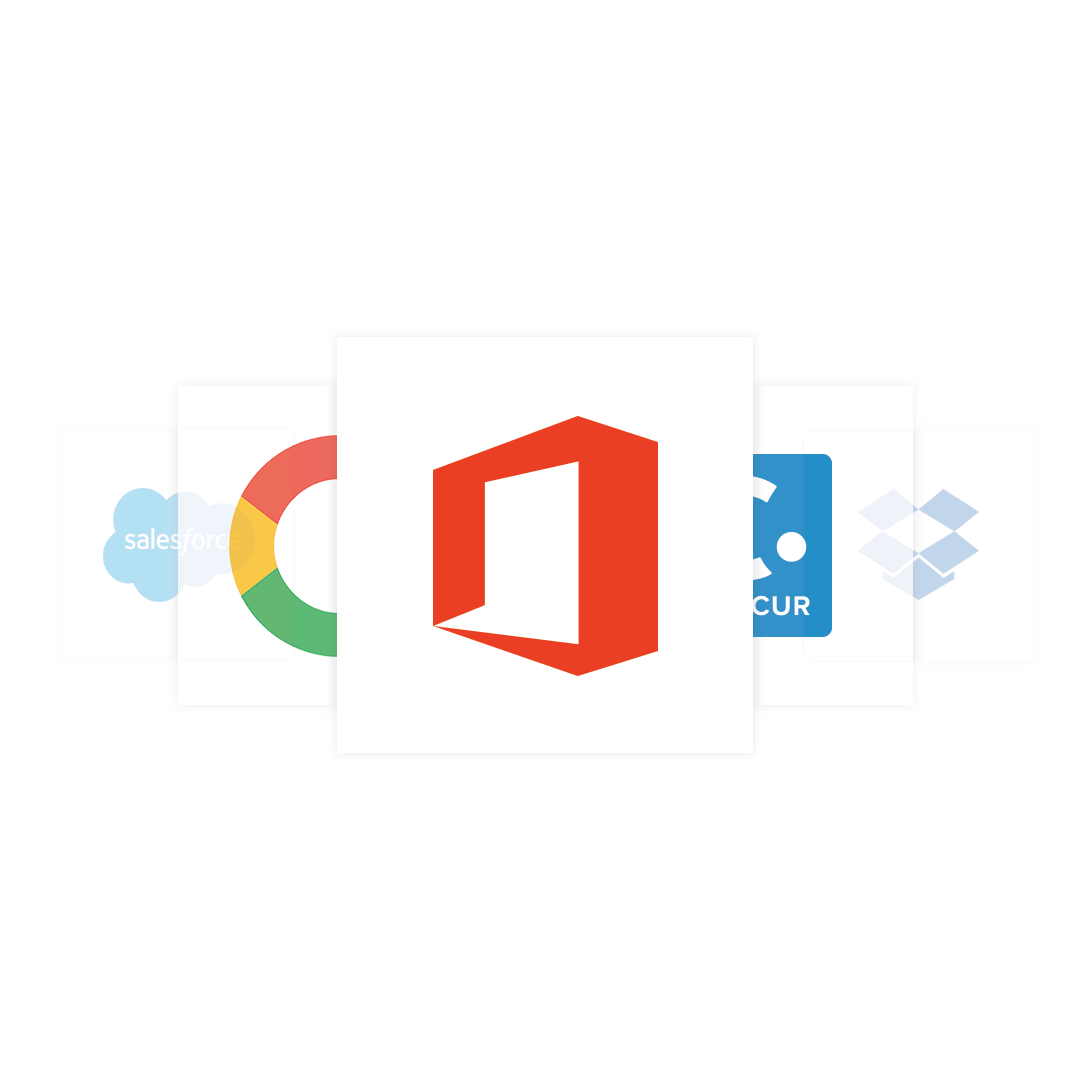The image features a visually intricate design against a stark white background, divided into three distinct layers composed of white squares. 

In the first layer, there is a prominent red 3D square box resembling the old, boxy television sets of the 1970s, lending a nostalgic vibe. Below this, part of the middle layer is visible, consisting of two red boxes over white squares, though only partially seen, hinting at their concealed design. On the left-hand side of this layer, a semi-circular shape is segmented into three horizontal stripes of red, yellow, and green, adding a splash of vibrant colors. On the opposite side, a blue square is seen with partial, enigmatic white text "C-U-R" and faint lines, suggesting a message or logo hidden from complete view.

The bottom layer, somewhat transparent, offers a glimpse of the earth or spherical design, enhancing the complexity of the composition. Finally, the left side of this layer features a blue cloud within a white square, symbolizing perhaps the sky or infinite possibilities, while the right side showcases an open blue box with a white interior, presenting a sense of openness and contrast.

The entire image merges contrasting colors and shapes, creating a dynamic and intriguing visual masterpiece.